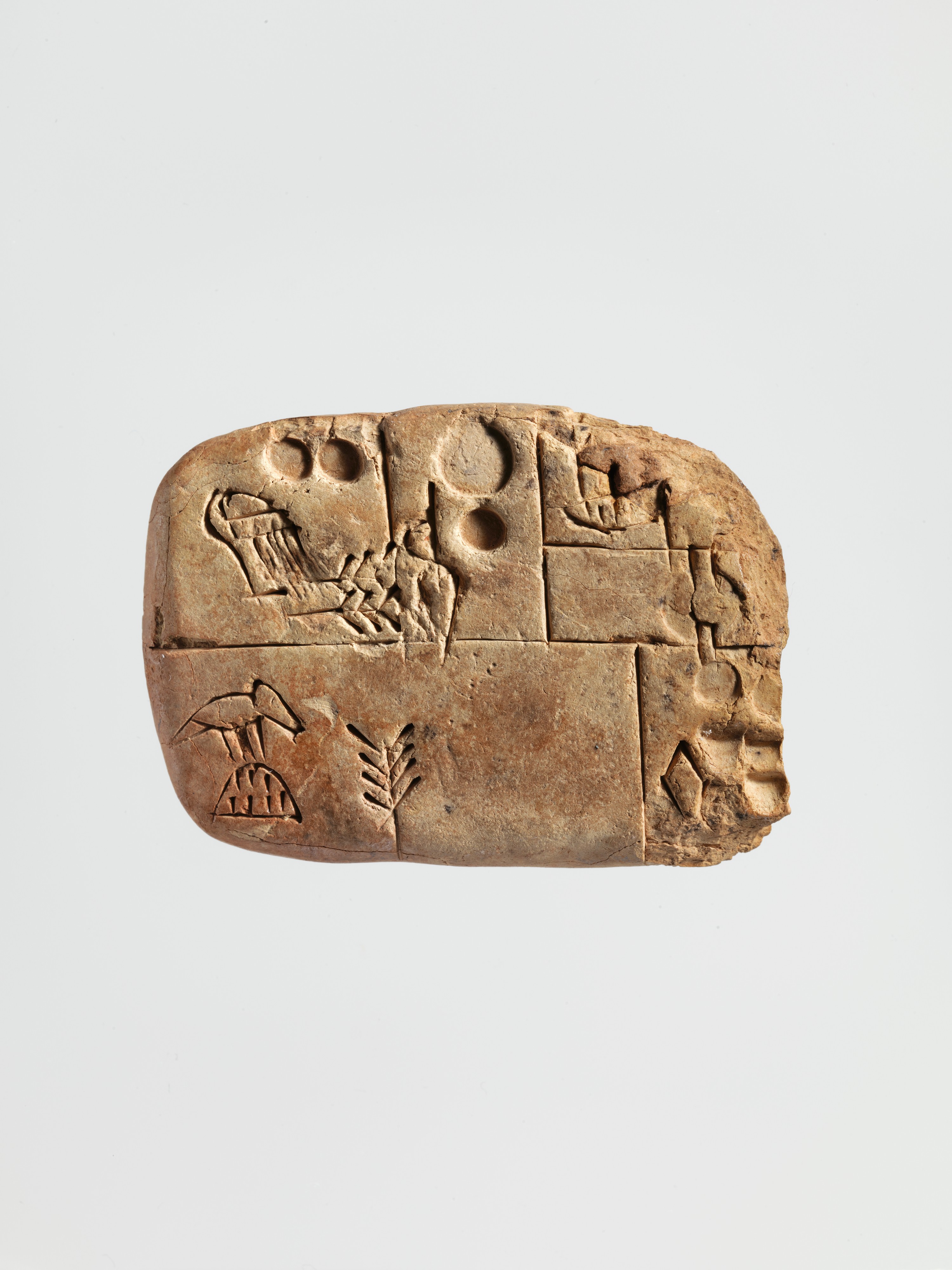The professional photograph, taken with excellent lighting, focus, and quality, showcases a rectangular piece of stone with soft, rounded edges, reminiscent of an archaeological find. Predominantly sand-colored with various shades of brown, the stone appears three-dimensional and ancient, potentially dating back thousands of years, possibly prehistoric or pre-biblical times. The surface of the stone is etched with intricate designs and divided into five distinct sections by horizontal and vertical lines. 

Prominently featured at the lower section of the stone is a depiction of a bird or possibly a dog-like animal standing on a hill, accompanied by what seems to be plant life, perhaps wheat or barley, characterized by straight lines with additional lines branching off. Other sections contain more abstract and difficult-to-interpret etchings, including small and large circles, jagged lines, and diamond shapes. Some areas have indentations as if made by a thumbprint. Despite the detailed artwork, there is no text accompanying the images. The overall appearance of the stone, with its detailed and mysterious engravings, strongly suggests it is an artifact of significant historical and cultural value.